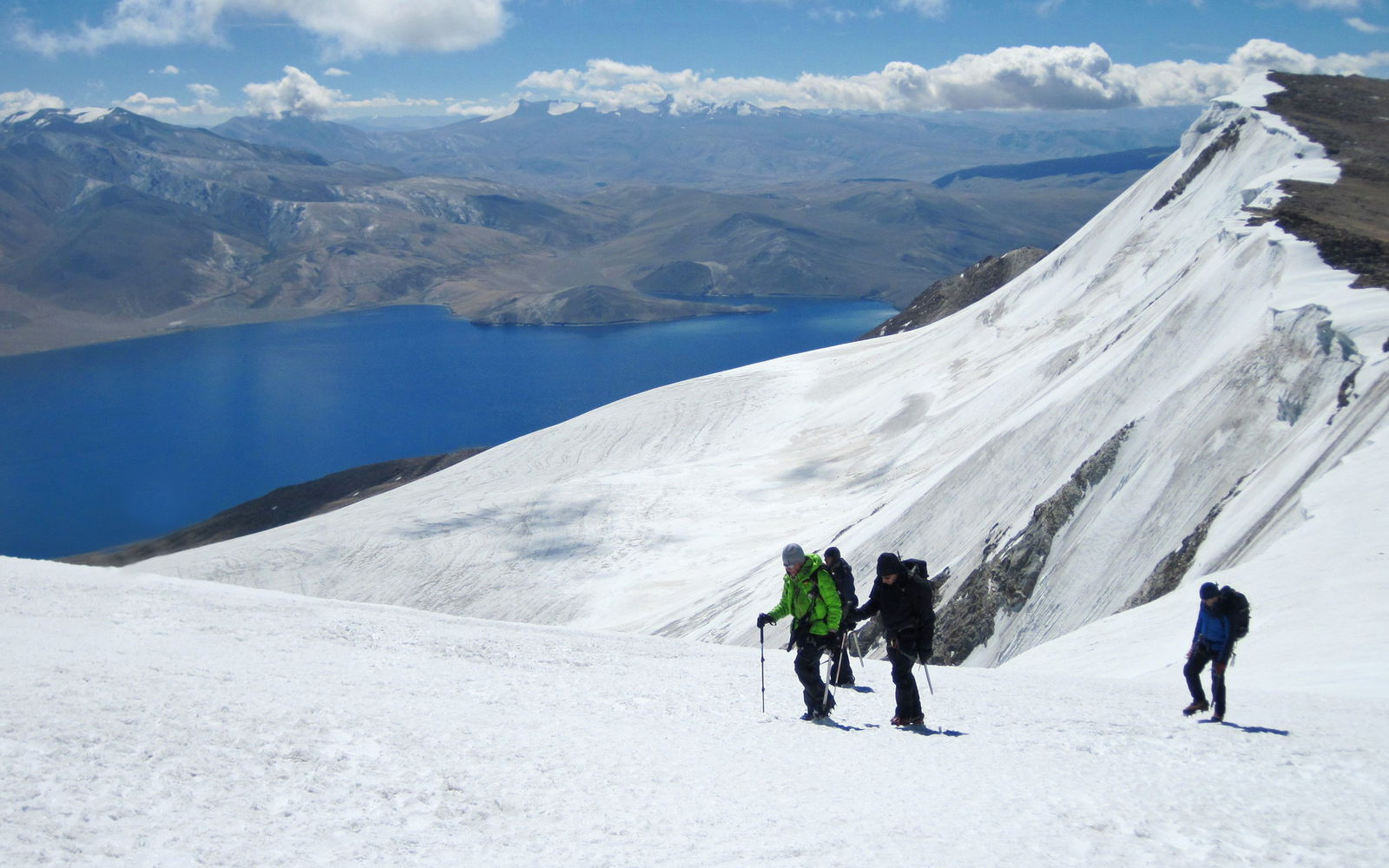The image features a group of four skiers, adorned in colorful ski jackets—green, blue, and black—and equipped with ski poles, making their way uphill on a snowy mountain slope. The foreground showcases the steep, ascending terrain they are navigating, possibly for skiing or snowboarding. In the distance, a sunny and cloudy sky presides over a vivid blue body of water, flanked by hills with snow-capped peaks. The background also displays a sharply descending slope devoid of people, enhancing the sense of solitude and adventure. Fluffy white clouds further decorate the sky, completing the picturesque scene of an alpine landscape.